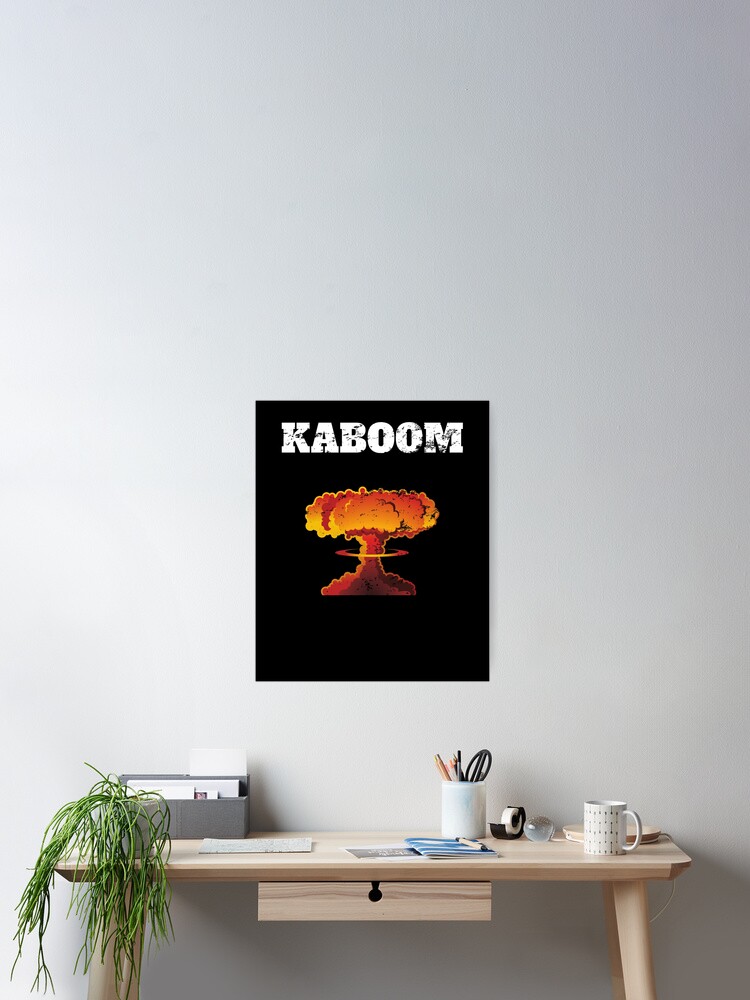This photograph captures the interior of a modern office room, highlighting a sleek, light wood-colored desk positioned at the bottom center of the image. The desk, contemporary in design and almost white in tone, is adorned with a variety of items that contribute to an organized and creative workspace. To the right, a bent, white desk lamp stands high next to a white coffee mug and a tape dispenser. Nearby sits a cup filled with scissors, pencils, and pens, while pamphlets lie in front. Dominating the left side of the desk is a small potted plant that resembles grass, placed in front of a gray paper storage box. Above this well-appointed desk, the eye is drawn to a striking black and orange poster affixed to the otherwise bare white wall. The poster, emblazoned with the bold text "Kaboom" at the top, features a vividly colored depiction of a nuclear explosion, with a mushroom cloud rendered in various shades of red, yellow, and orange. The overall setting reflects a stylish and meticulously curated work environment.